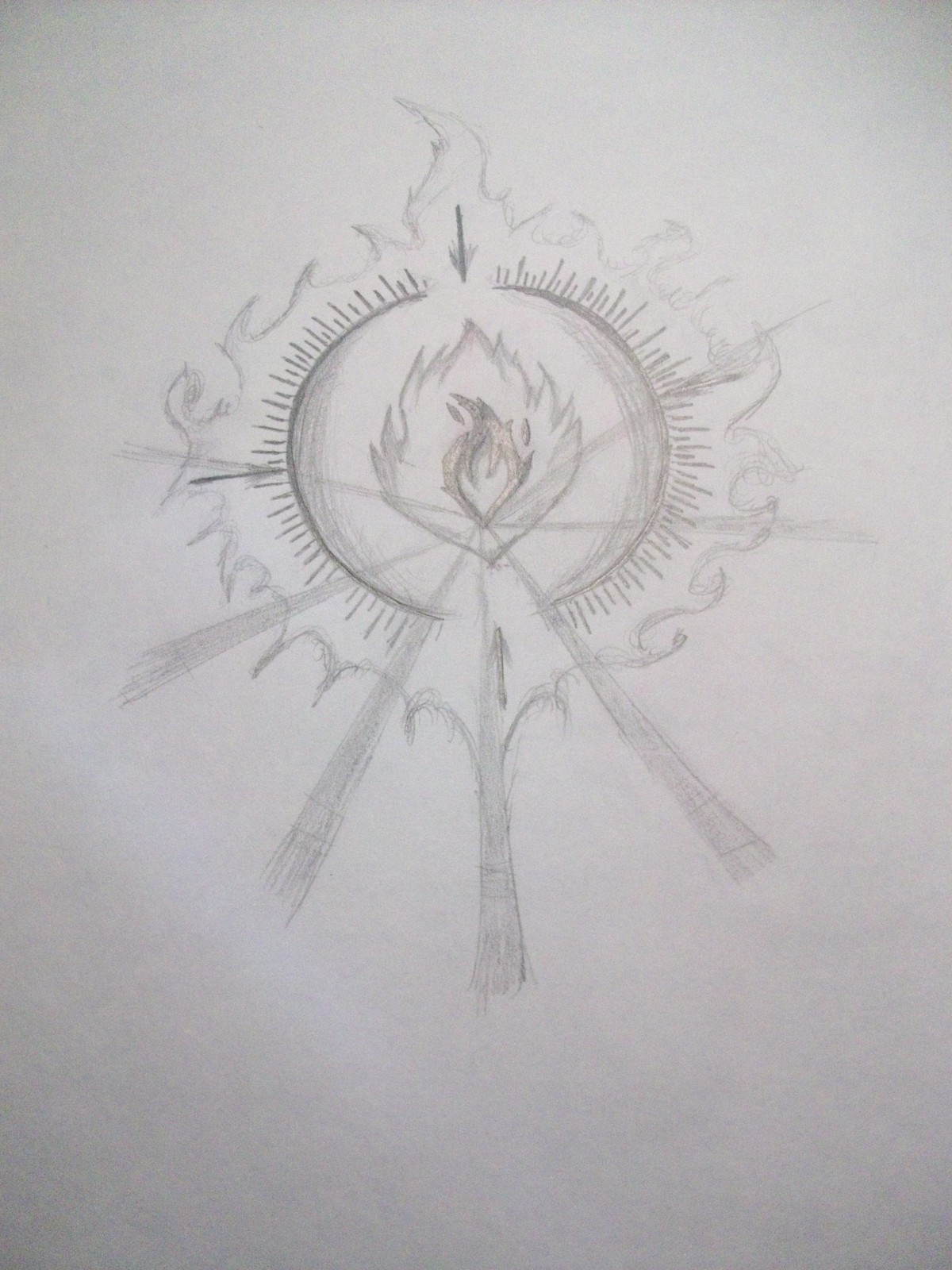The detailed pencil drawing portrays a flame at its center, encircled by intricate layers of additional flame-like lines. The main flame is nested within a smaller flame, with three arrows pointing inward from the outer edges toward the central blaze, creating a sense of focused energy. Surrounding the flames are delicate, radiating lines that extend outward from the center, emulating rays of light and enhancing the depiction of the flame's intensity. Encasing the entire composition is a partially broken circle, with visible gaps at the top and bottom, which interacts with the outermost flames. The entire artwork, set against a white background, is richly shaded in pencil, using variations in line and shadow to convey the dynamic and radiant nature of the flame.